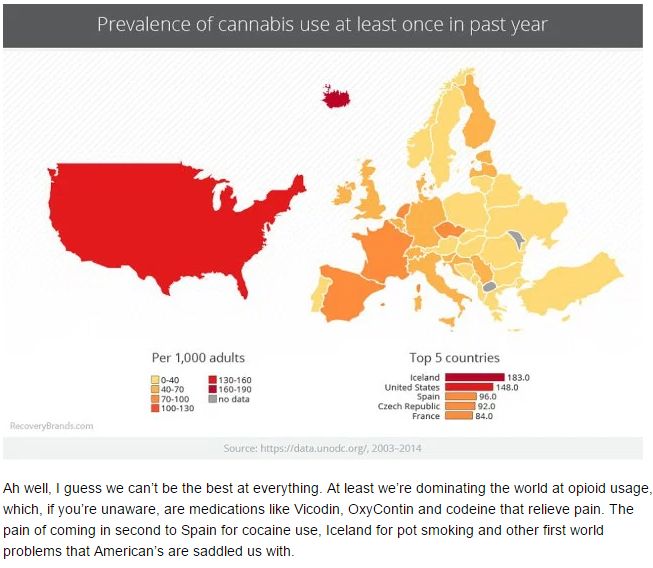This image is an informational chart depicting the prevalence of cannabis use in multiple countries, focusing on Europe and the United States. At the top, a dark grey horizontal stripe contains the title in light grey text, "Prevalence of Cannabis Use At Least Once in Past Year." Below this, the chart features a red map of the United States on the left and a color-coded map of Europe on the right, representing cannabis usage rates per 1,000 adults. The color key, ranging from light yellow (0-40) to dark red (160-180), with grey indicating no data, is provided for clarity.

On the right side, the chart lists the top five countries for cannabis use: Iceland (183.0), United States (148.0), Spain (98.0), Czech Republic (92.0), and France (84.0). Beneath these rankings, black text humorously comments, "Ah, well, I guess we can't be the best at everything. At least we're dominating the world at opioid usage, which, if you're unaware, are medications like Vicodin, Oxycontin, and Codeine that relieve pain. The pain of coming in second to Spain for cocaine use, Iceland for pot smoking, and other first world problems that Americans are saddled with." The background of the image is predominantly white, making the graphical elements and text stand out effectively.